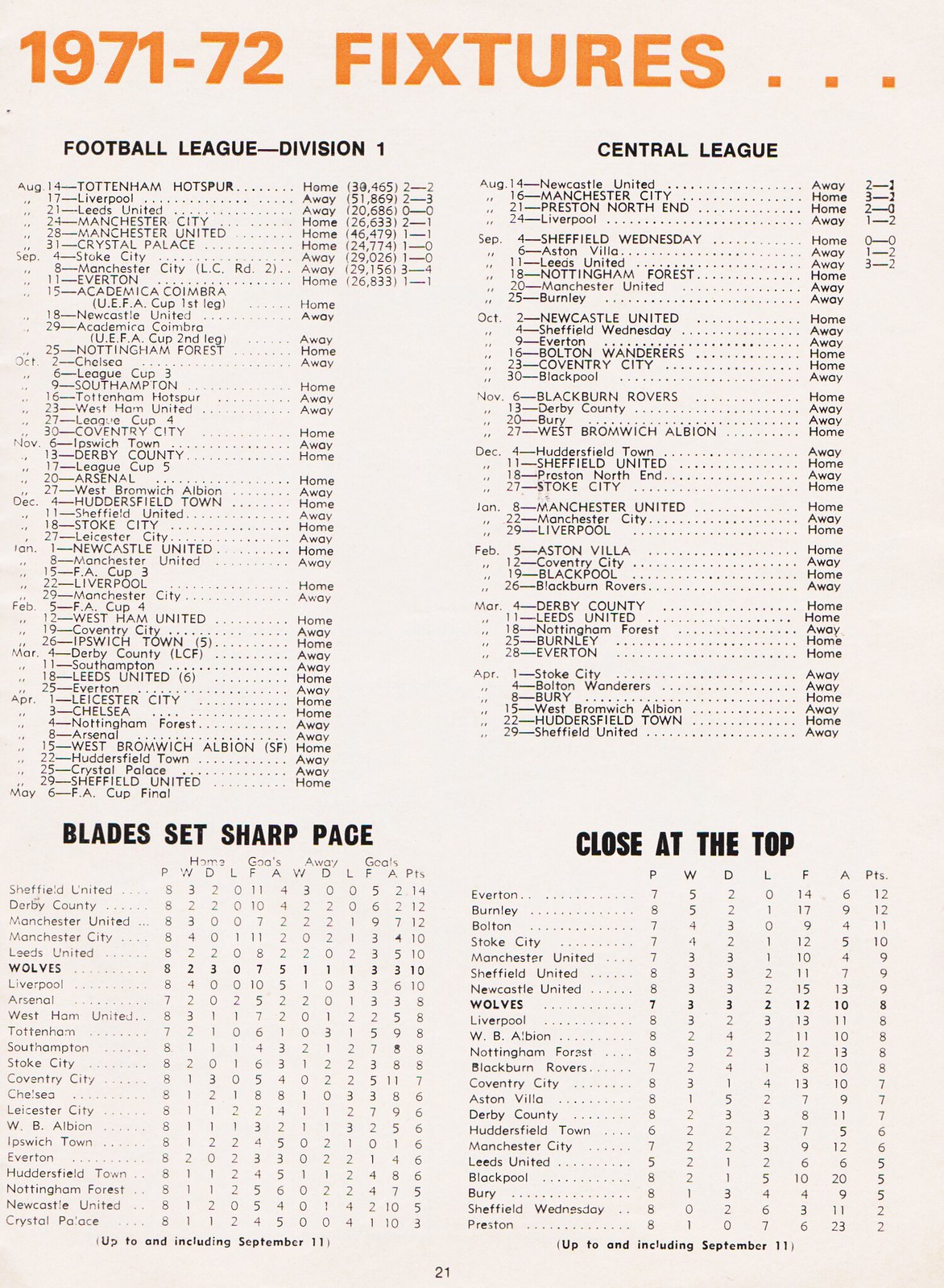The image is a promotional document for a football league, prominently featuring the text "1971 to 1972 Fixtures..." in bold orange, all-caps font at the top against an off-white background. Below this header, the page is divided into four distinct categories, each with its own table of information in black text. 

In the top left corner, the "Football League Division I" section lists various teams along with their respective home and away matches, organized by month. Notable teams include Tottenham Hotspur (highlighted as the author's favorite), West Ham United, Huddersfield Town, and West Bromwich Albion, with notable match dates starting from August 14th.

The top right corner houses the "Central League" section, which similarly details teams and their match schedules, organized by month.

The bottom left section, labeled "Blades Set Sharp Pace," provides further information on different teams, while the bottom right section, titled "Close at the Top," continues to list team-specific details.

Noteworthy visual details in the image include Wolves (presumed to be Wolverhampton) bolded within the tables, and "Page 21" indicated at the very bottom of the page. The entire document is in black and white, except for the striking orange header.